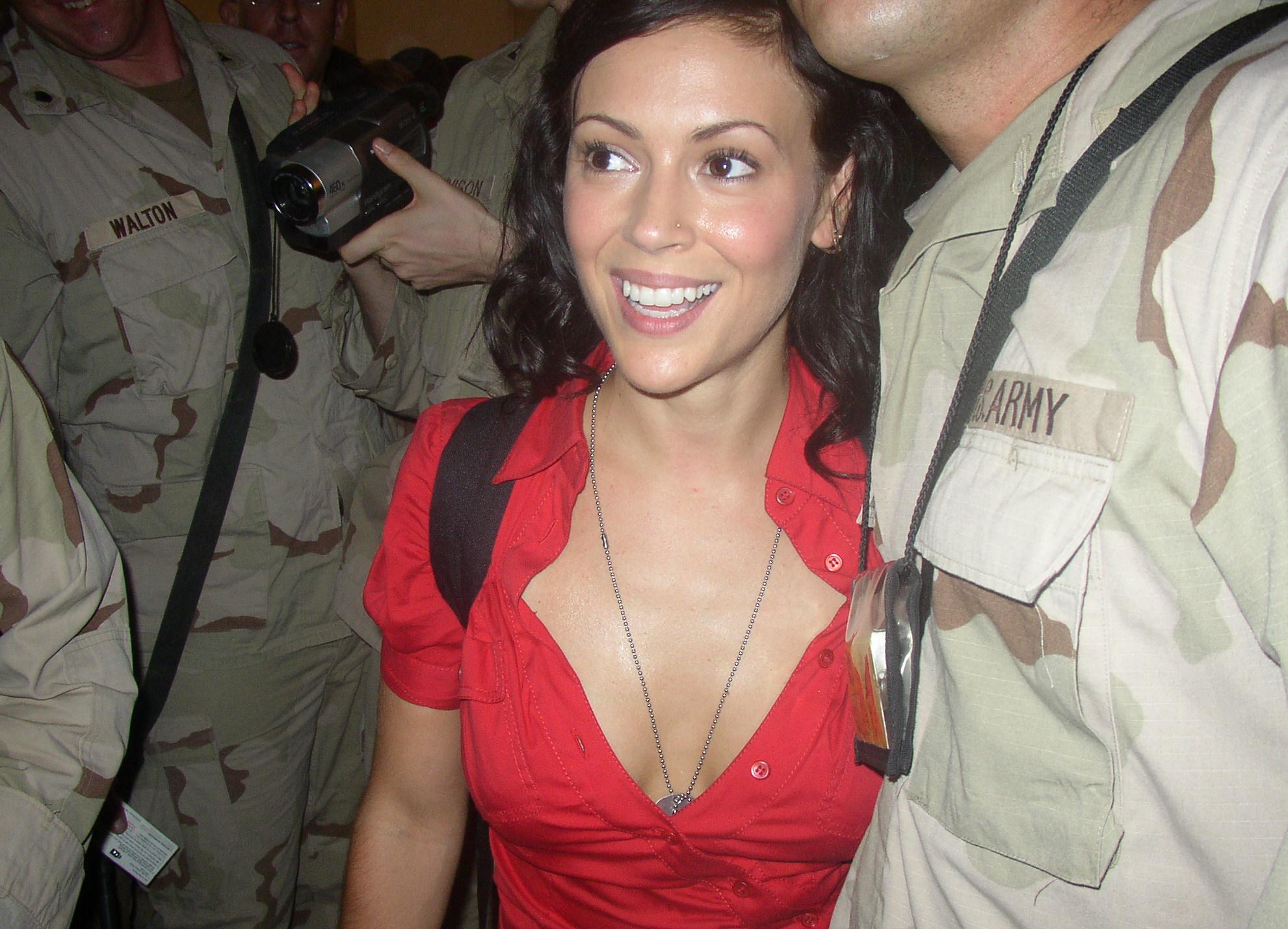In this photograph, actress and model Alyssa Milano is at the center of a group of army soldiers in camouflage uniforms of green, brown, and tan. Milano is wearing a low-cut red button-up blouse that reveals a silver dog tag necklace draping down towards her chest. She has shoulder-length brown hair, thin black eyebrows, a nose piercing, and an ear piercing in her visible left ear. With a bright smile on her face, she appears to be looking towards another camera. She carries a backpack and is positioned at chin level to a taller soldier beside her, whose face is only partially visible with stubble on his chin. This soldier has a black strap pouch around his neck and an 'Army' label over his right breast pocket. To Alyssa's left, there are three more soldiers, partially obscured, with one bearing a nametag that reads "Walton." One of the soldiers nearby is holding a camcorder.